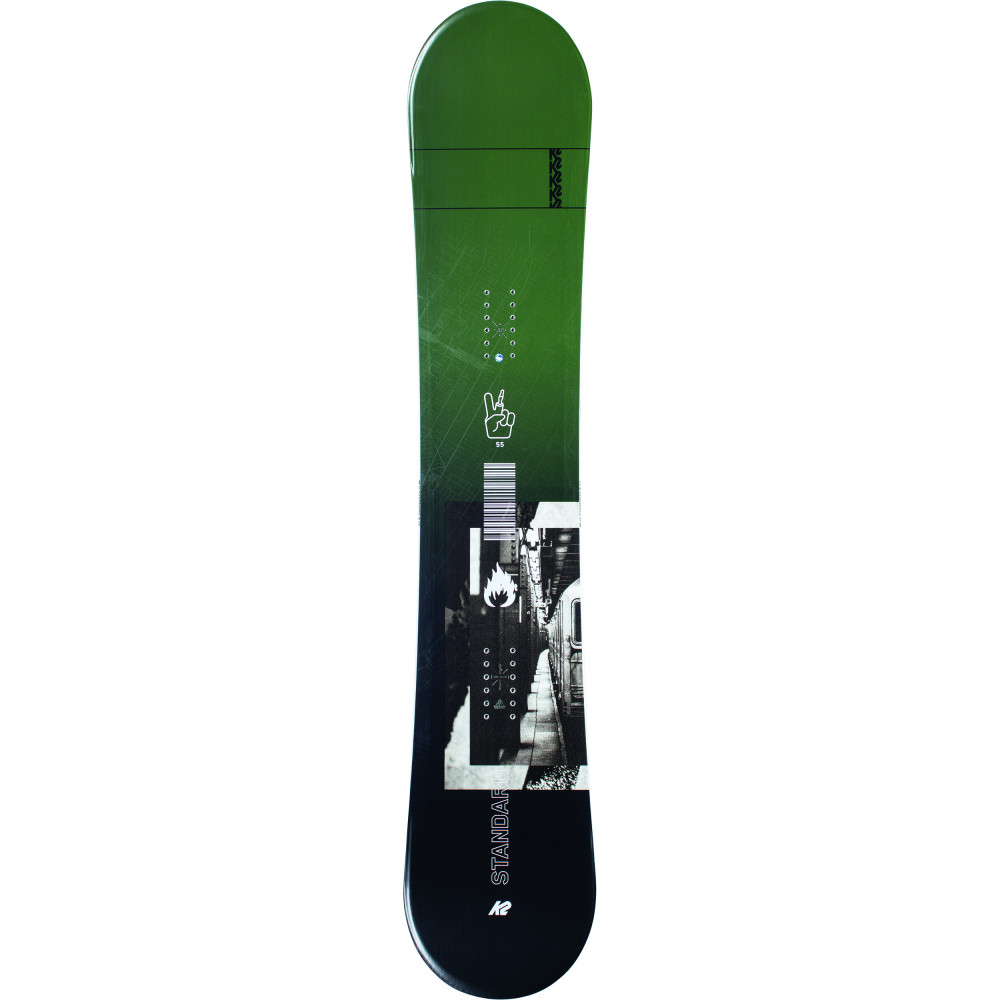This image is a detailed, color photograph with a portrait orientation, prominently featuring a single snowboard positioned vertically in the center against a completely white background. The snowboard has a shiny finish that transitions from olive green at the top to solid black at the bottom. It is visually striking due to its minimalistic yet bold color palette of green, black, white, and shades of gray. The upper half of the snowboard includes a white outline of a hand giving the peace sign, centered above a black and white illustration of a subway station corridor with visible train tracks. Below this illustration lies a barcode with a white flame above it. The word "standard" appears in typography on the side of the snowboard, though it is partly cut off and somewhat illegible. The sleek, edgy design and high-quality photographic style suggest that this image could be used on a sporting goods website.